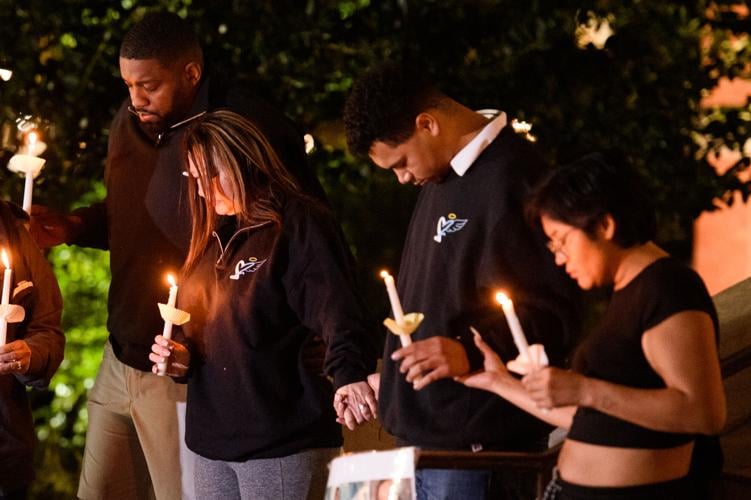The photograph captures a somber candlelight vigil held outdoors, with four prominent individuals in the foreground set against the backdrop of green trees and grass. All four participants have their heads bowed and eyes closed, deeply immersed in a shared moment of remembrance. Each person holds a lit white candle, symbolizing unity and reflection.

Starting from the left, the first individual is an African American man dressed in a dark shirt and khaki pants, with his head lowered as he holds a lit candle in his right hand. Beside him stands a woman with long brown hair, wearing a dark shirt featuring a heart and winged angel logo, and gray athletic pants. She grips the hand of the next individual, an African American man, who also wears a similar dark shirt with jeans. His head is bowed while holding the woman's hand with his right hand and a candle in his left. The fourth individual, a woman with short hair and glasses, is dressed in a cropped black t-shirt and holds a candle in her left hand while clinging to the arm of the man next to her with her right hand. The group's attire and the candles they hold reinforce the vigil's solemn atmosphere, underlining the collective sense of mourning and solidarity.